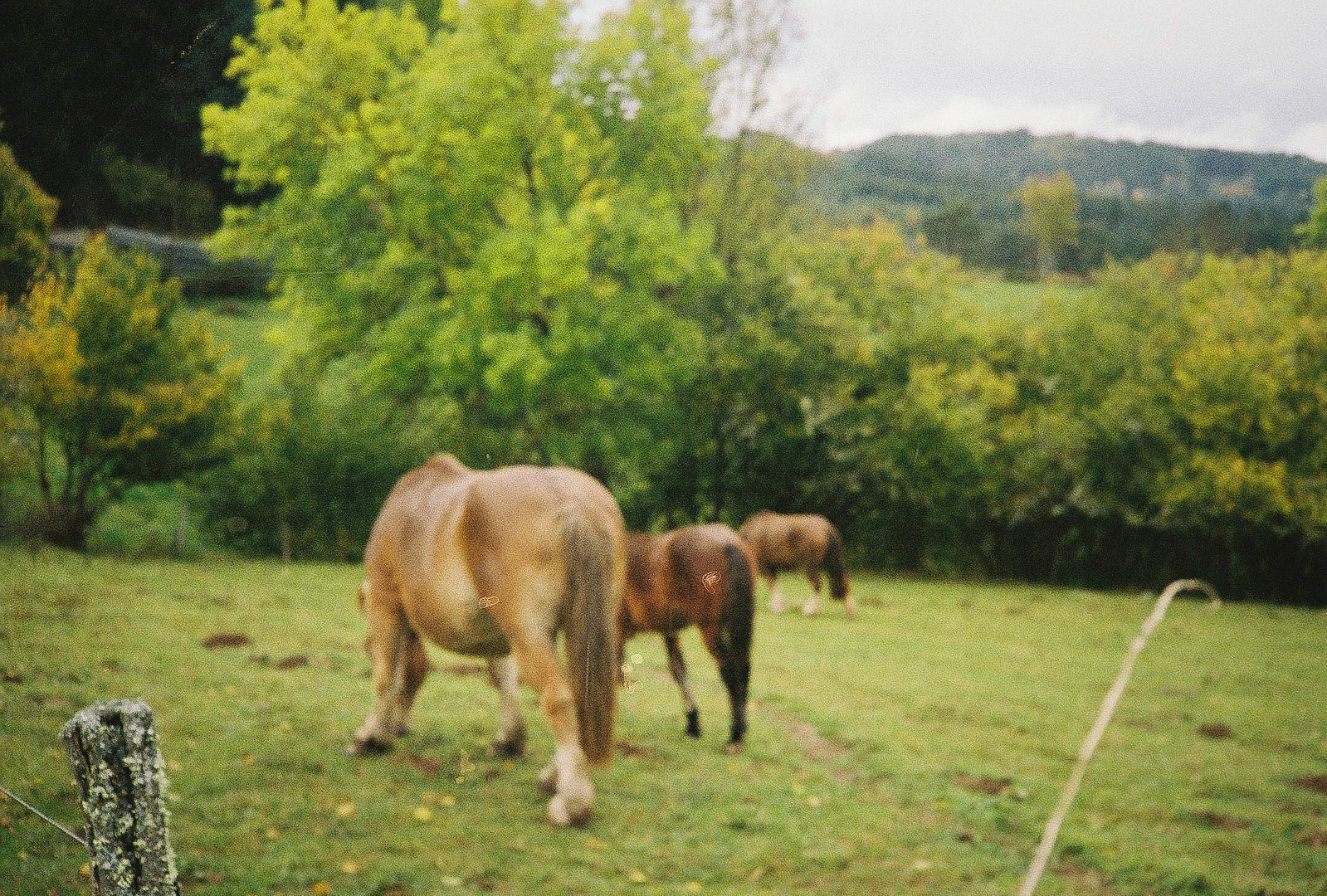In this grainy photograph, three brown horses stand in an open pasture, all facing away from the camera with their heads lowered to graze on grass. The horse on the left appears to be the lightest in color, the middle one the darkest, and the one in the background an in-between shade. The terrain is inclined, with patches of bare dirt and scattered yellow leaves. A thin, somewhat flimsy fence is indicated by a post on the bottom left with a line trailing from it. In the background, the landscape features green and light green bushes and trees, with dense tree coverage making the upper left corner particularly dark. Farther back on the right side, hills can be seen in the distance beneath a hazy blue and white cloudy sky. The overall image quality may be low, but the pastoral scene is still discernible.